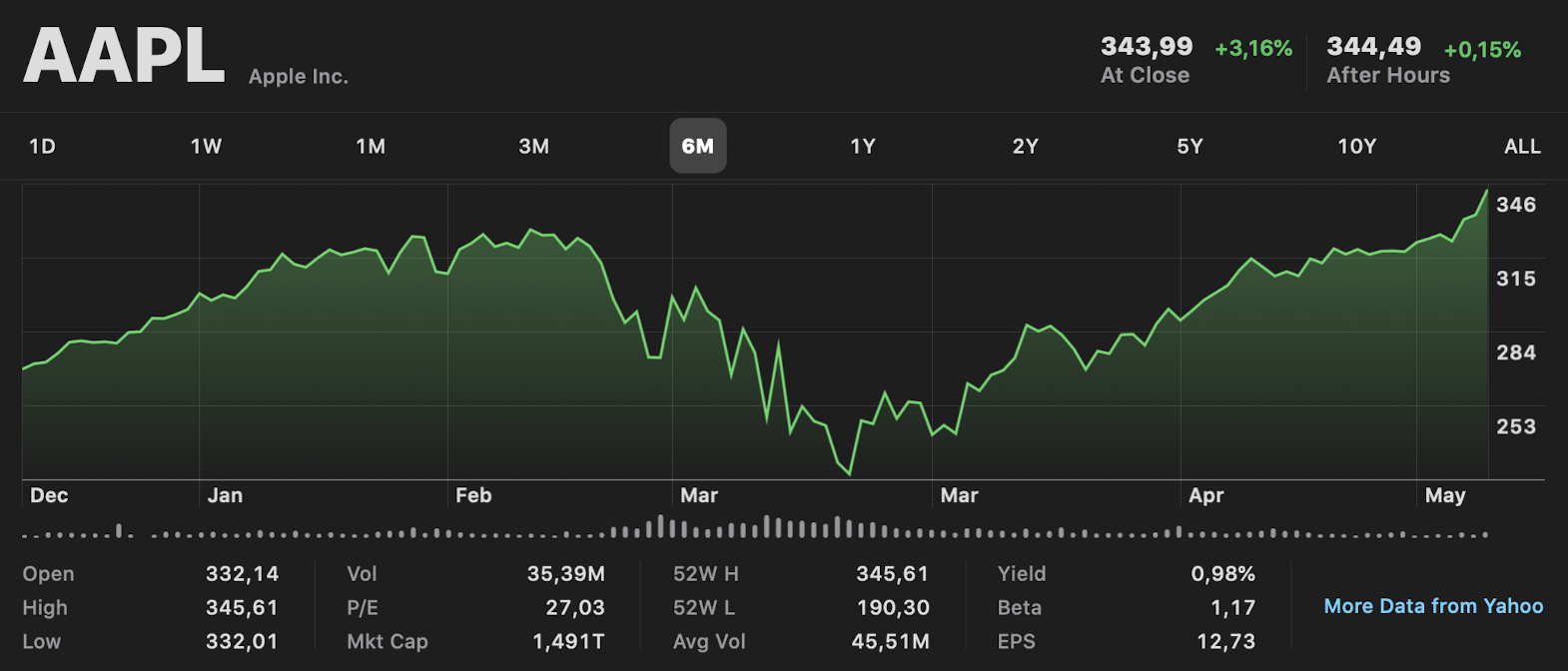A detailed and cleaned-up caption for the given image could be:

"The image portrays a stock chart for Apple Inc. (AAPL). At the top left, the label 'Apple Inc.' is displayed, alongside its stock symbol 'AAPL.' In the upper right corner, key financial figures are present: '344.49' next to '+0.15%' in green, and below this in gray, 'After Hours.' To the left, '343.99' is displayed next to '+3.16%' in another green figure, with 'At Close' indicated underneath in gray text. 

The stock chart itself is depicted with light green lines, while the area beneath these lines has a green tint. Along the bottom right, 'More data from Yahoo' is written in light blue text. The x-axis of the chart from the mid-left to mid-right shows the months, labeled as December, January, February, March, April, and May. In the bottom left corner, various data points for the chart such as 'Open,' 'High,' 'Low,' 'Volume,' 'P/E,' and 'Market Cap' are shown, providing further insights into Apple's stock performance."